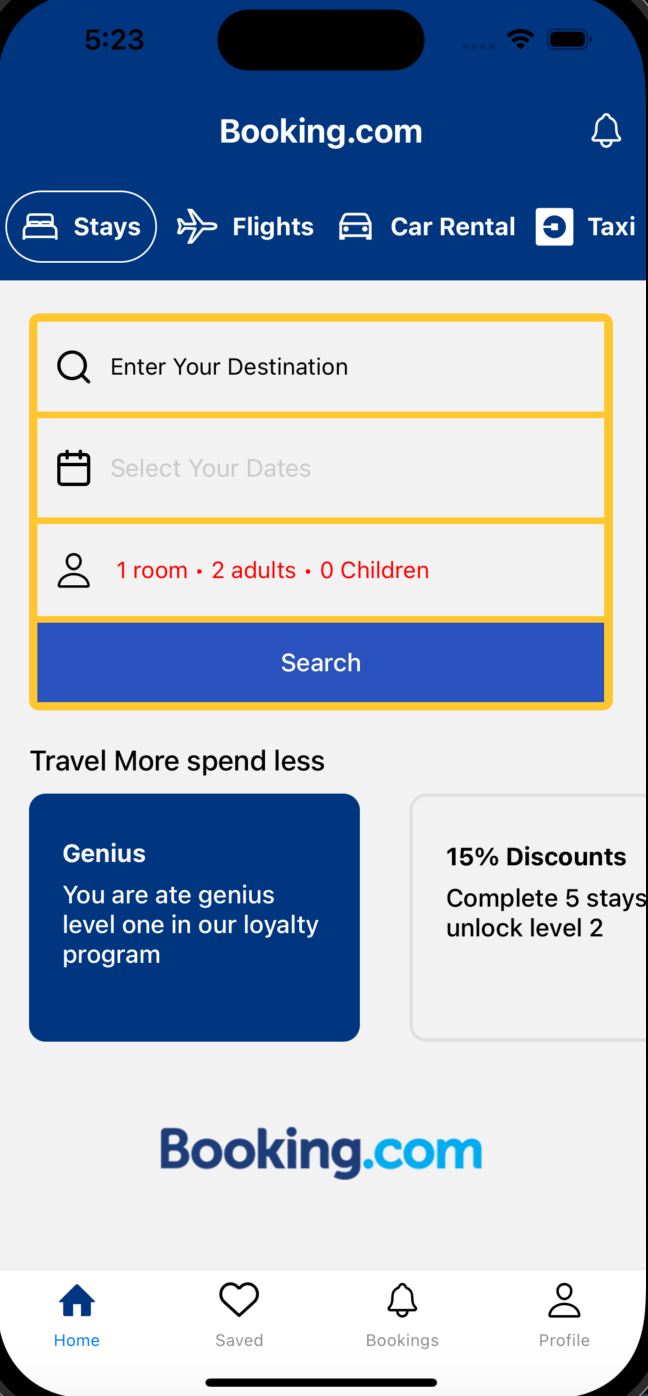This is a highly detailed screenshot from the Booking.com mobile app displayed in portrait mode. The user interface features a primarily blue and white color scheme with the Booking.com logo prominently displayed near the bottom of the screen. Along the bottom row, there are navigation icons labeled Home, Saved, Bookings, and Profile. At the very top, the screen displays the title "Booking.com" with a notification bell icon adjacent to it. Just below the title, there are tabs for Stays, Flights, Car Rental, and Taxi, with the "Stays" tab currently selected.

The main content area starts with a couple of form fields. The first field, marked by a magnifying glass icon, prompts the user to "Enter Your Destination." The second field, indicated by a calendar icon, is for selecting dates and labeled "Select Your Dates." Below these fields, an icon of a person signifies room and occupancy details, displaying "One Room, Two Adults, Zero Children" in red text. Encased within a yellow-bordered box, the prominent blue "Search" button resides below these fields, inviting the user to submit their selections.

Beneath this form, a blue-bordered informational section reads "Travel More, Spend Less." Within the section, it notes, "This is Genius. You are a genius, level one in our loyalty program." Adjacent to this is another box highlighting a 15% discount offer, with the text: "Complete five stays, unlock level two." It is noteworthy that within the first box, there is an error stating "you are eight genius" instead of the intended "you are a genius."

The entire setup provides a user-centric interface designed for easy navigation, emphasizing user loyalty benefits while guiding travelers seamlessly through the booking process.